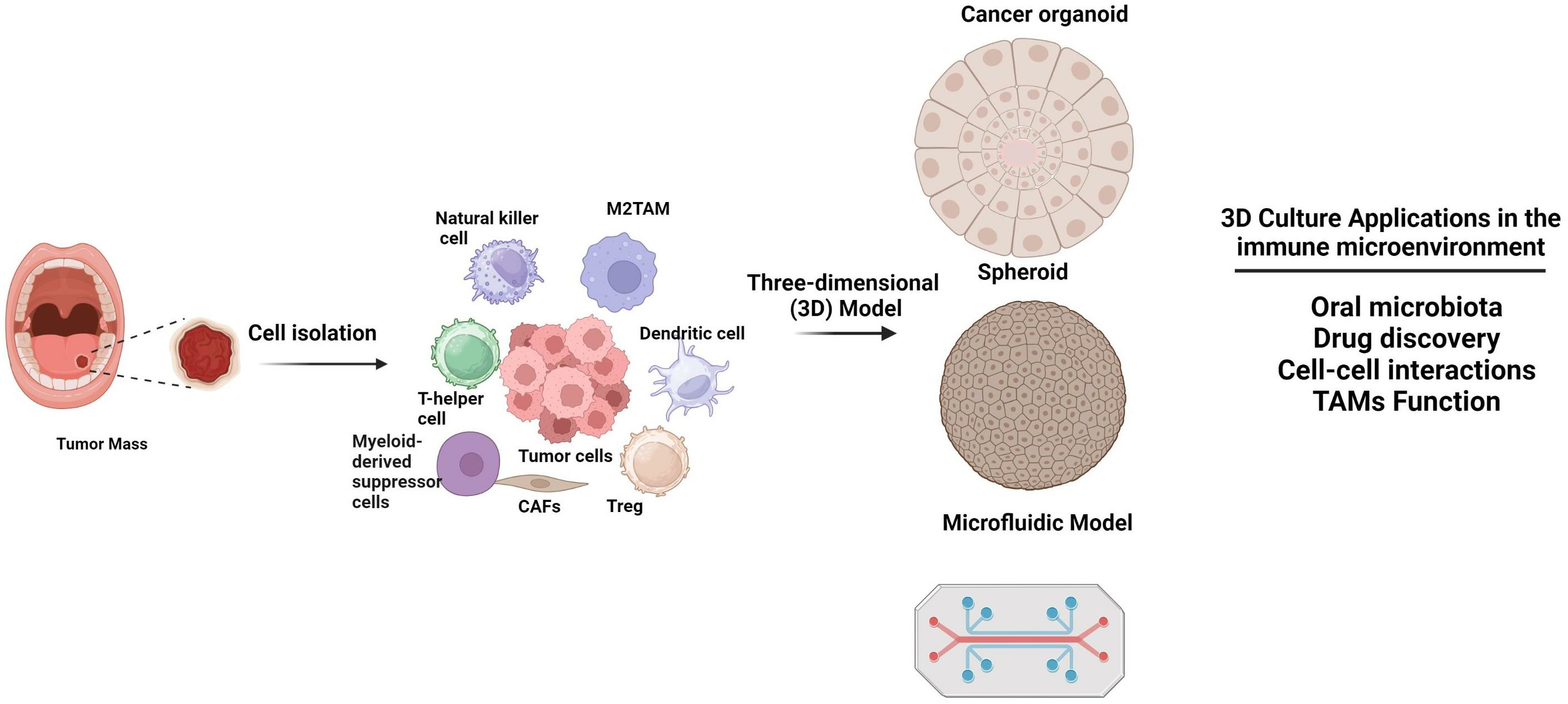The image is a detailed anatomical and cellular diagram on a plain white background, roughly six inches long and three inches high. On the far left, an open mouth is depicted, exhibiting a tumor mass on the right side of the tongue. The mouth illustration includes the teeth, tongue, epiglottis, and throat. Labeled "tumor mass," a red dot on the tongue indicates the tumor’s location, leading to a larger, magnified visual of the tumor as a jagged red circle. 

To the right of this, the diagram is labeled "cell isolation," featuring an arrow pointing towards various colored cells, including a green T helper cell positioned between a blue natural killer cell and purple myeloid-derived suppressor cells. Additional cells such as M2TAM, dendritic cells, TREG, tumor cells, and CAFs are also presented.

Further to the right, the label "three-dimensional 3D model" introduces a detailed representation of a cancer organoid, depicted as a light brown sphere with embedded cells, and a microfluidic model, illustrated as a dark brown solid sphere with cellular structures. Another section resembling a circuit board is also shown.

At the bottom right, the caption reads "3D culture of applications in the immune microenvironment," followed by a list: oral microbiota, drug discovery, cell-cell interactions, and TAMs function. The diagram integrates detailed labels and arrows, providing a comprehensive visual representation of the tumor microenvironment and associated cellular interactions.